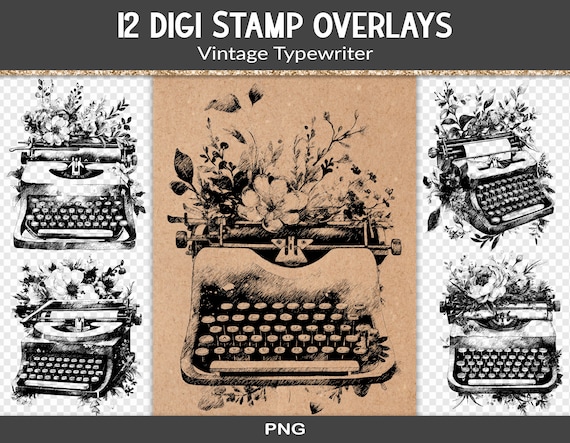The image is a set of graphics depicting vintage typewriters, creatively designed with plants and flowers emerging from them. At the top, the text reads "12 DigiStamp Overlays Vintage Typewriter," suggesting these are digital stamps meant for overlays, created on a computer. In total, there are four typewriters displayed in various styles and angles, each adorned with large, blooming flowers. The leftmost typewriter appears old, with plants growing out of it, while the one below it looks even more antiquated, also with plants sprouting from the top. In the middle, a typewriter features an elevated carriage with flowers emerging around it. The two typewriters on the right continue this floral theme, integrating flowers prominently into the design. The text is presented in white on a black background, and at the bottom of the image, there is the acronym “PNG,” indicating the file format.